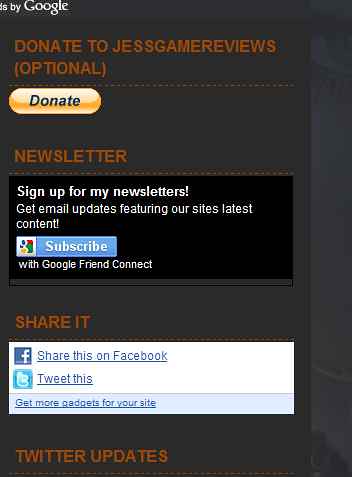The image is a detailed screenshot from a mobile phone browser displaying a charity donation page for "JazzGamerReviews." The background of the page is primarily gray and charcoal. At the top, there is an orange text that reads "Donate to JazzGamerReviews," accompanied by a prominent donate button. Below this section, there's a newsletter signup prompt, offering the latest content updates via email. The subscribe button is white and blue. Further down, there's a "Share It" banner with red letters on a gray background, providing options to share the page on social media platforms such as Facebook and Twitter. Additionally, the text mentions "Twitter updates" and "Get more gadgets for your site" towards the bottom. This comprehensive setup is formatted for easy navigation and interaction on a mobile screen.